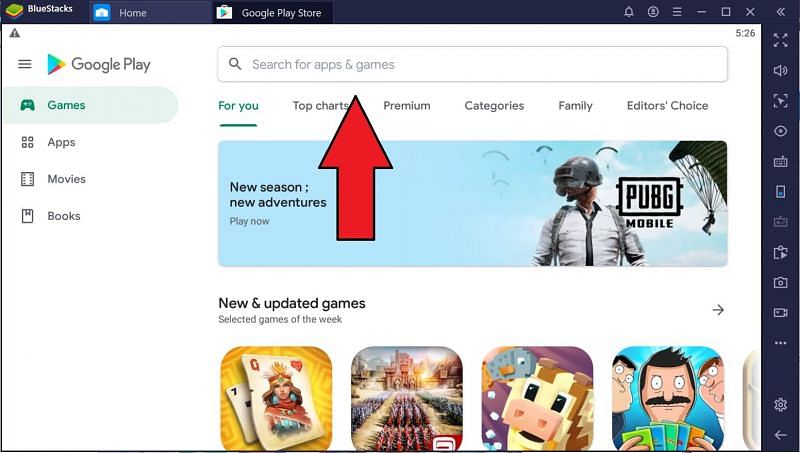The image depicts an older version of the Google Play Store as displayed on the BlueStacks emulator. Dominating the top of the screen is a navy blue border extending around the top and right side. At the top-left corner, the BlueStacks icon is visible, followed by a navigation menu featuring "Home" and "Google Play Store."

Beneath the BlueStacks header, the typical Google Play side menu is displayed, showcasing categories such as Games, Apps, Movies, and Books, each accompanied by corresponding icons. In the center of the image, a prominent search bar labeled "Search for apps & games" is followed by a menu laying out several options: For You, Top Charts, Premium, Categories, Family, and Editor's Choice. A notable red arrow points between the "Top Charts" and "Premium" categories, leading to an advertisement dominating the center of the screen.

The advertisement, set within a light blue box, promotes the game "PUBG Mobile," heralding a new season and new adventures. The ad features an illustration of a man wearing a VR headset, skydiving with a parachute, rendering an adventurous theme. Below this ad, on a white background, is the "New & Updated Games" section, highlighting the games of the week.

Displayed under this section are images of four games:
1. A game featuring playing cards, possibly solitaire.
2. A game involving soldiers and a castle.
3. An animated game with a cow, suggesting some type of farming game.
4. An image of Peter Griffin from Family Guy with his friends, seemingly playing poker.

On the right side within the navy blue bar are several icons related to the Google Play Store functionalities, including notifications, an X for closing, speaker, and camera icons.